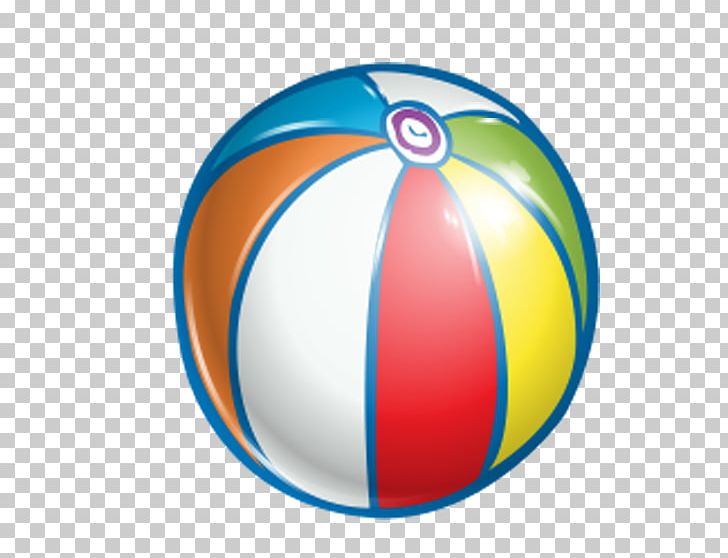In this digital image, created likely for use as an icon in web design or presentations, there is a single object prominently featured: a beach ball. This beach ball is positioned directly in the center of a checkered background pattern composed of grey and white squares, which indicates transparency in digital images. The artistic style is cartoony and somewhat childish, suggesting a playful beach volleyball setting.

The beach ball itself is outlined in blue and exhibits multiple vibrant colors arranged in a segmented pattern reminiscent of banana shapes. Starting from the top, the central button-like circle displays a white and purple color scheme. Radiating from this central point, the segments of the beach ball display the following sequence of colors: blue, orange, white, red, yellow, another segment of orange, and then white again. Each segment is bordered in blue, enhancing the vividness of the colors, which include turquoise, green, and contrasting shades of blue. The overall design is playful and visually appealing, making it suitable for digital media that aims to convey a fun, beach-like atmosphere.